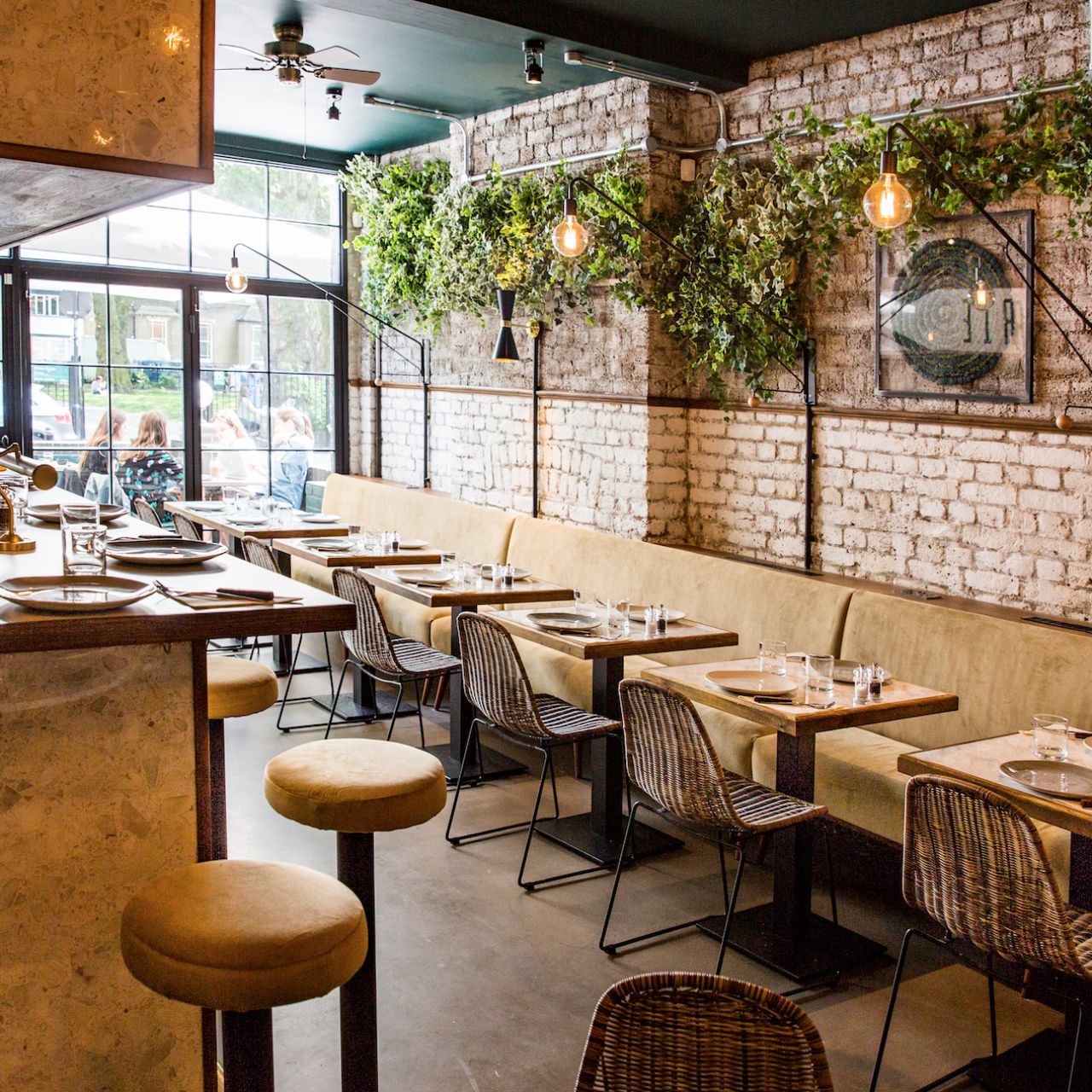This photograph captures the inviting interior of a restaurant bathed in daylight, with seating areas both inside and outside. Inside, the arrangement includes six square dining tables, flanked by sturdy, fabric-made twine chairs on one side and tannish-colored booth seating along a brick-colored wall adorned with lush green plants and foliage, giving the space a vibrant, earthy vibe. The restaurant features a back wall with a stone facade, partially cloaked in ivy-like greenery, contributing to the organic and neutral aesthetic. Above, black industrial-style lighting fixtures with Edison bulbs hang, casting a warm glow over the seating areas. Ceiling fans offer respite on warmer days. 

A bar with approximately five high-top gold-colored bar stools is positioned near the front, defined by glass walls with black framing, suggesting a modern yet cozy atmosphere. The building is situated in a mixed residential and business area, indicated by the presence of houses visible across the street and patrons enjoying their meals outside. The entirety of the restaurant's design, from the earthy tones to the thoughtfully placed greenery, speaks to a harmonious blend of nature and contemporary comfort.